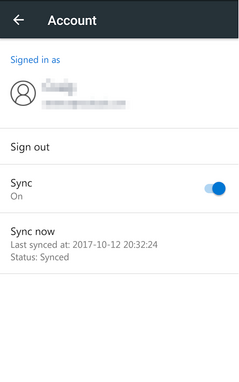A user is navigating their account settings on an Android phone. The screen displays a section titled "Signed in as," where the name and email have been blurred out for privacy. The profile picture slot is empty, showing a default silhouette of a person. There is a "Sign out" button available twice on this page. 

One setting labeled "Sync" can be toggled on or off; in this case, it is toggled on. Another option labeled "Sync now" allows immediate synchronization instead of regular intervals. The last sync occurred on October 12th, 2017, and the status indicates the sync is complete.

The overall design of the page is minimalistic with a white background. The top section, where "Account" is written, has a black background with white text. A back arrow next to "Account" presumably leads to more general settings.